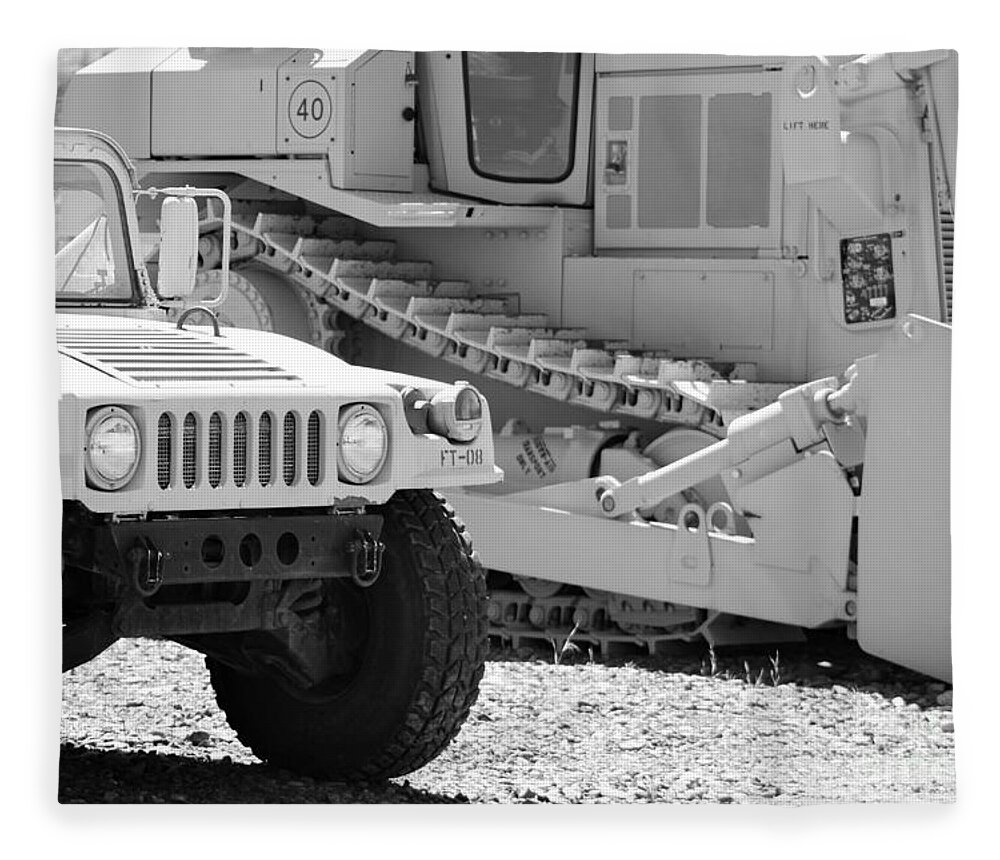In this black and white photograph, the viewer is presented with a rugged scene featuring heavily weathered industrial and military equipment situated in a dirt field or possibly an overgrown grass lot. The image is in landscape orientation, evocative of an old, almost timeless quality due to the lack of color. To the left side of the photograph, a portion of a military Humvee is captured, showcasing its angled front grille, two distinct round headlights, and a single, hefty tire with pronounced treads. The vehicle's windshield and a sizeable side mirror add to the visibility of its utilitarian design. Just behind the Humvee, another formidable piece of machinery, possibly a bulldozer or an earth mover, is partially seen. This equipment is marked with the number "40" and features large tracks that dominate the viewer's perspective. Although faded and barely discernible, text like "FT-08" and other notations hint at the machine's robust, operational past. Both vehicles appear to be in similar hues of light gray to near white, blending slightly with the desaturated landscape. The composition suggests a still and abandoned environment, likely a training ground, where the once-powerful machines now rest in silent repose.